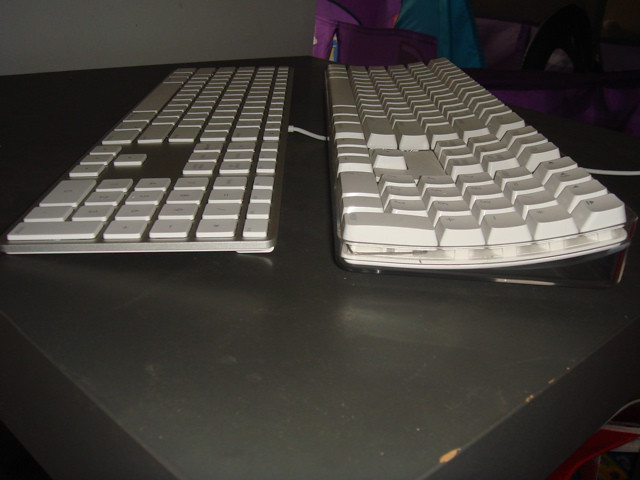The image shows a rectangular gray table with noticeable scratches on its right side, set against a dark, poorly lit background. The table appears to have a pointed front and back, creating an elongated, diamond-like shape. Two white keyboards are placed vertically on the table, with the left keyboard being a sleek, flat Mac keyboard, distinguished by its shallow, squared keys and a cord that extends out of the picture. The right keyboard has more pronounced, elevated keys, suggestive of an older design, and features a subtle curvature in the middle. Behind the table, the background is somewhat blurred and dark, showing indistinct shapes and colors, including red, pink, blue, and purple, potentially indicating a person wearing a multicolored jacket or shirt, but details are unclear due to the poor lighting.